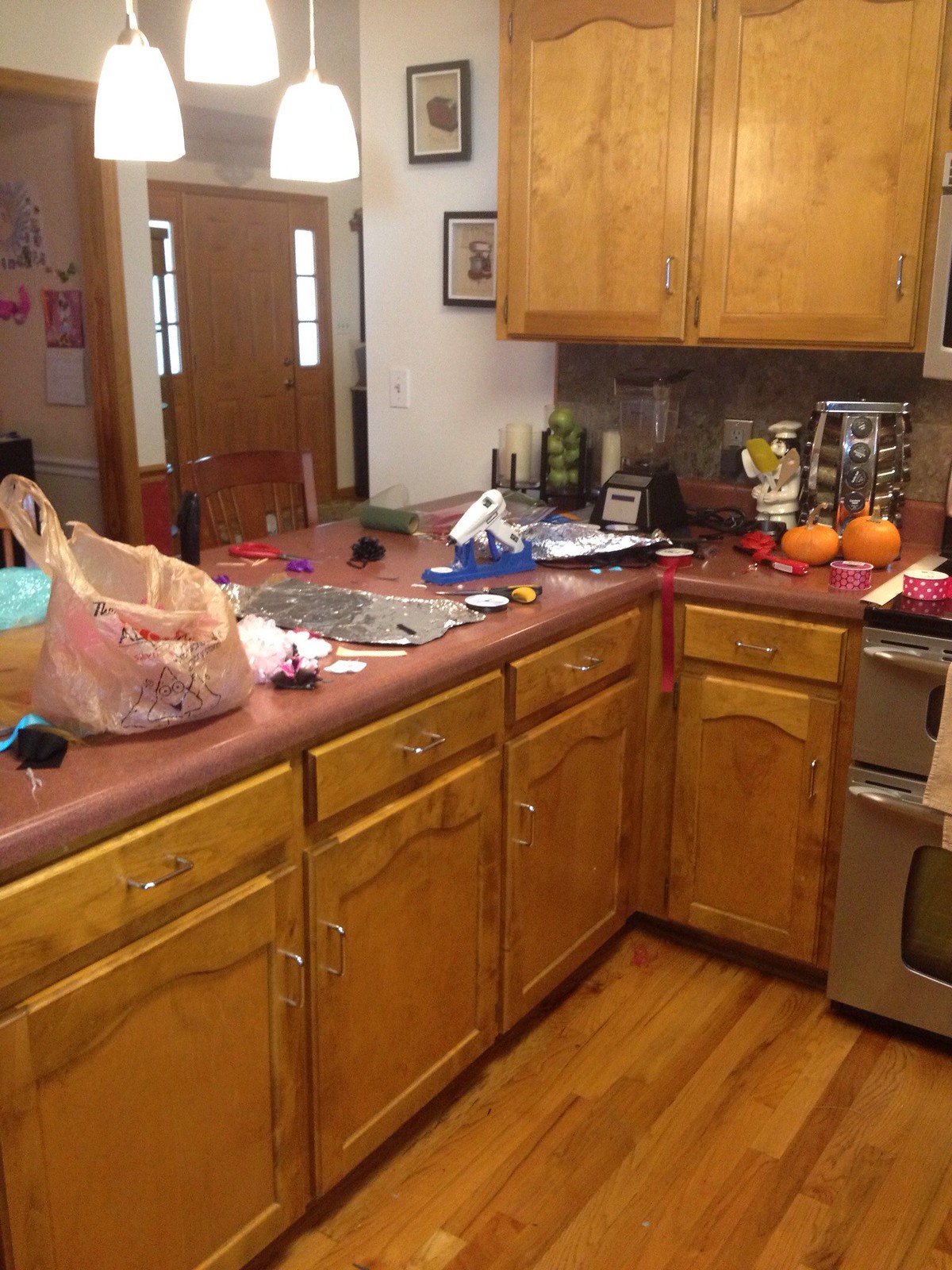The photo captures the interior of a cozy kitchen, with the image oriented towards the left of a stainless steel stove. The focal point, however, is the array of kitchen cabinets to the left of the stove, made of rich brown wood and adorned with sleek silver pull handles. The countertop beneath these cabinets is a pinkish laminate, creating a subtle contrast with the dark wood and the variety of objects arranged atop it.

Starting from the right, adjacent to the stove, there is a sleek, silver rotating spice rack filled with an assortment of spices, introducing a touch of culinary readiness. Sitting nearby are a couple of vibrant orange citruses, adding a pop of color to the scene. A charming painted statue of a chef stands proudly, injecting a bit of whimsy and personality into the kitchen ambiance.

Continuing leftwards, a modern blender with a black and white base occupies its spot, plugged into a wall outlet, ready for action. Adjacent to it, a cluster of green apples rests in a black holder, evoking a sense of freshness and health. Spread out along the flat part of the countertop is a piece of foil and a brown plastic bag, indicative of recent or upcoming food preparation. Adding a playful element, a small child's toy, colored pink and black and equipped with roller wheels, sits on the counter, hinting at a family-friendly environment.

The kitchen floor, composed of brown wood matching the cabinets, extends its warmth throughout the space, unifying the overall aesthetic of this inviting kitchen.